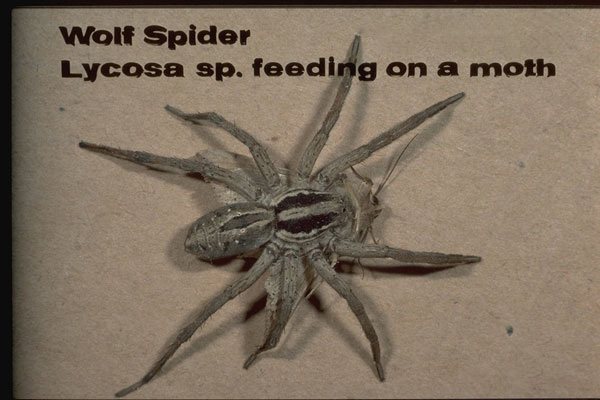This is a highly detailed photograph of a wolf spider, specifically identified as Lycosa SP., feeding on a moth. The top of the image displays text in black bold lettering that reads "wolf spider Lycosa SP. feeding on a moth." The spider, seen from an overhead view and facing right, is situated on a solid surface that is either concrete or gray cardboard, exhibiting a grayish or tan color. The spider itself is significant in size, roughly comparable to a human hand, with a large, thick body and long, slightly furry legs.

The spider's coloration encompasses various shades of gray, adorned with distinctive black markings and two prominent black stripes running down the front portion of its body. Its back features three horizontal stripes, resembling stitches on a football. The spider casts a shadow on the surface due to its size and the lighting in the photograph.

Beneath the spider, the outlines of a moth are visible, with its wings protruding from underneath the spider’s legs and its tentacles peeking out near the spider’s mouth. The details of this predatory scene, combined with the spider's intricate markings and imposing appearance, create a striking and somewhat unsettling image, highlighting the raw aspects of nature.